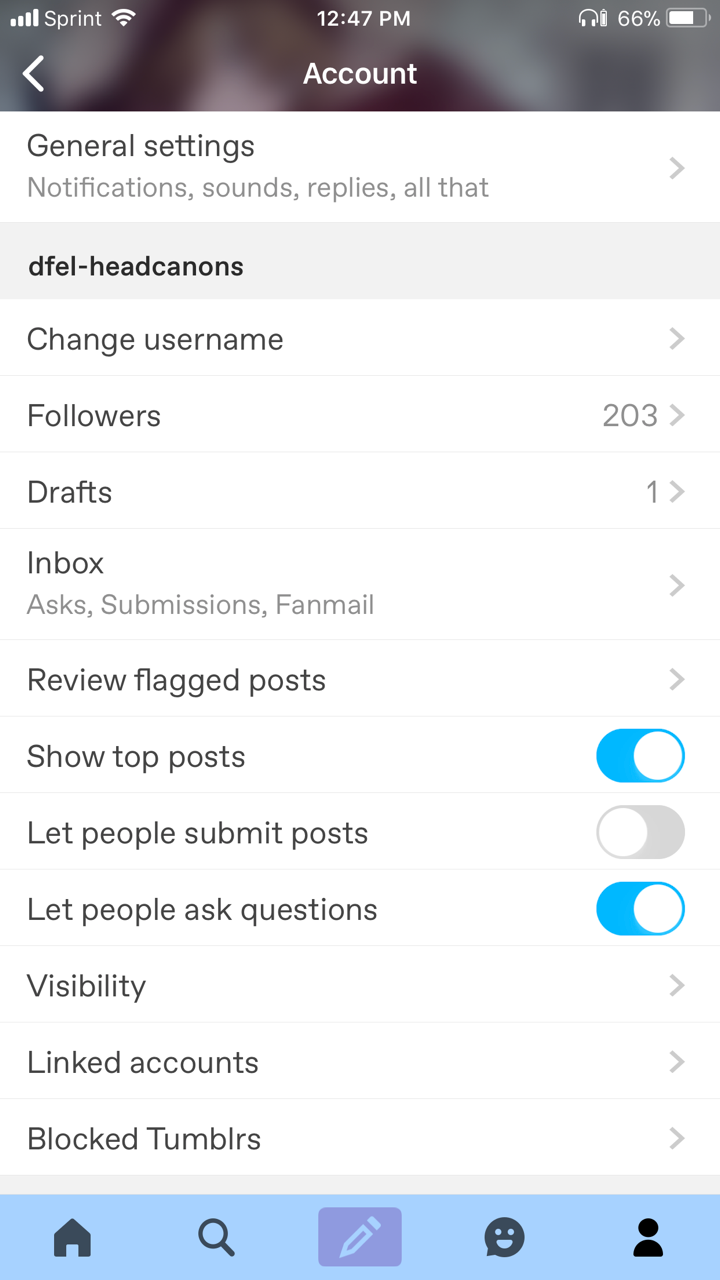A vertically-oriented smartphone screenshot, likely from an iPhone or an Android device, is displayed. The topmost part of the image is slightly blurry, featuring a dark rectangle filled with various status icons and information.

- **Status Bar:**
  - **Top Left:** Four out of four signal bars indicating strong network connectivity.
  - **Next to Signal Bars:** The carrier name "Sprint".
  - **Next to Carrier Name:** A Wi-Fi symbol.
  - **Next to Wi-Fi:** The current time shown as "12:47 p.m." in white letters.
  - **Top Right:** A row of icons including a headphone symbol, an unfamiliar white icon, a battery percentage at 66%, and a three-fourths filled battery icon.

- **Content Below Status Bar:**
  - Directly below the signal bars is a sideways arrow (V) pointing left.
  - **Middle of the Screen:** A white rectangular area displaying in black text "General Settings". Below this title are menu options in light gray text, including "Notifications," "Sounds," and "Replies," with a rightward-facing gray arrow next to each.
  
- **Menu Options:**
  - A slim gray bar with black text reading "DFEL - Head Cannons".
  - Below this, text in black displays "Change Username" with a sideways gray V pointing right.
    - Each menu section is delineated by faint gray lines.
  - Under "Change Username" is "Followers" followed by the number 203 and a sideways gray V.
  - "Drafts" is listed next, showing the number 1 and a gray V.
  - The "Inbox" option follows, with subcategories "Asks," "Submissions," and "Fan Mail" in gray text, accompanied by a gray V.
  - "Review Flagged Posts" appears next with a gray V.
  
- **Toggle Settings:**
  - "Show Top Posts" features a toggle switch currently set to on, indicated by a blue oval with a white circle on the right.
  - "Let People Submit Posts" has a grayed-out toggle switch with the white circle on the left (off position).
  - "Let People Ask Questions" includes a blue toggle switch indicating it is on (white circle to the right).
  
- **Additional Options:**
  - "Visibility" is listed with a gray arrow pointing right.
  - "Linked Account" has a similar gray arrow.
  - "Block Tumblrs" also features a gray arrow.
  
- **Bottom of the Screen:**
  - A thin gray line precedes a large light aqua-blue bar containing five icons from left to right:
    - A black house icon (likely Home).
    - A magnifying glass icon (Search).
    - A purple rectangle with a pencil icon (Compose).
    - A speech bubble with a smiley face (Messages).
    - A black person icon (Profile).